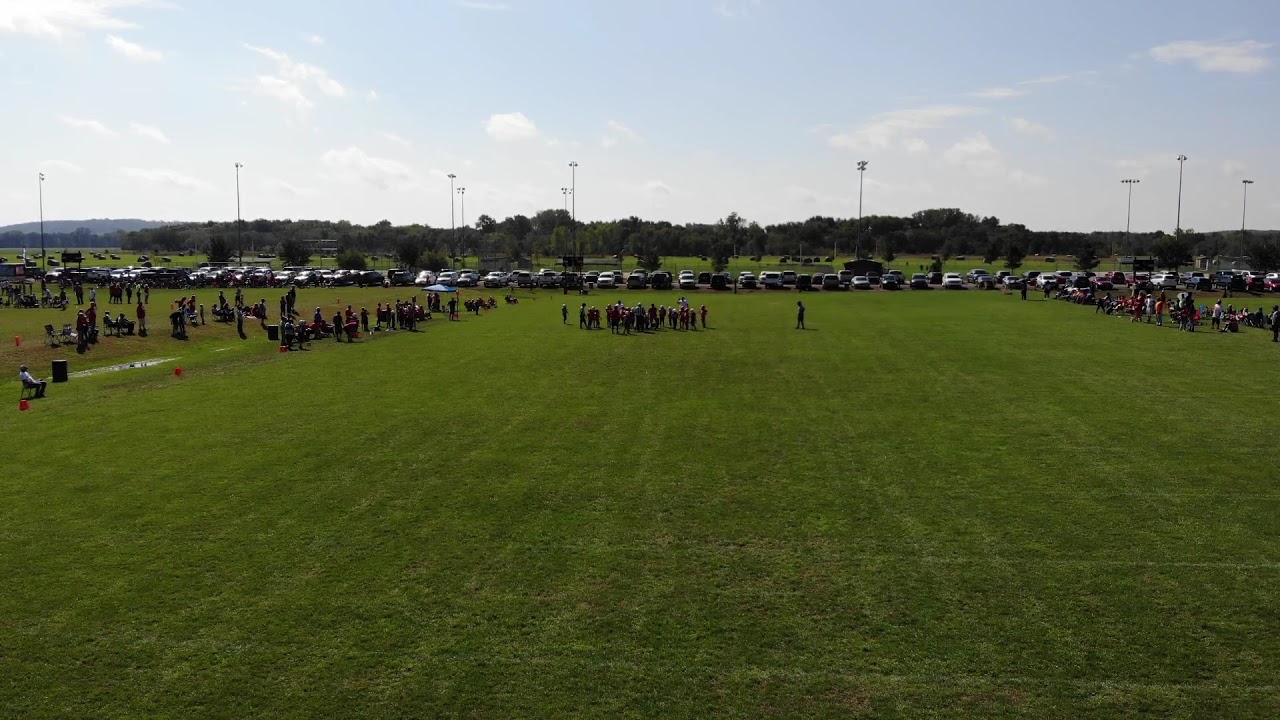The image depicts a lush green grass field, which appears to be a football or soccer field, captured from an aerial perspective, likely by a drone. Dominating the center of the photograph is a group of people gathered around what seems to be a coach, suggesting a sports event or practice session. Smaller clusters of spectators are visible on the left and right sides of the field. In the background, a long row of cars is parked, with tall street lights positioned between the parking area and the field. Beyond the cars, a dense line of dark green trees stretches across the horizon, accompanied by a distant mountain on the left side. The sky above is a very light blue, adorned with wispy and puffy white clouds, enhancing the serene atmosphere of the scene. Orange cones are set up on the left side of the field, further indicating an organized sporting activity.